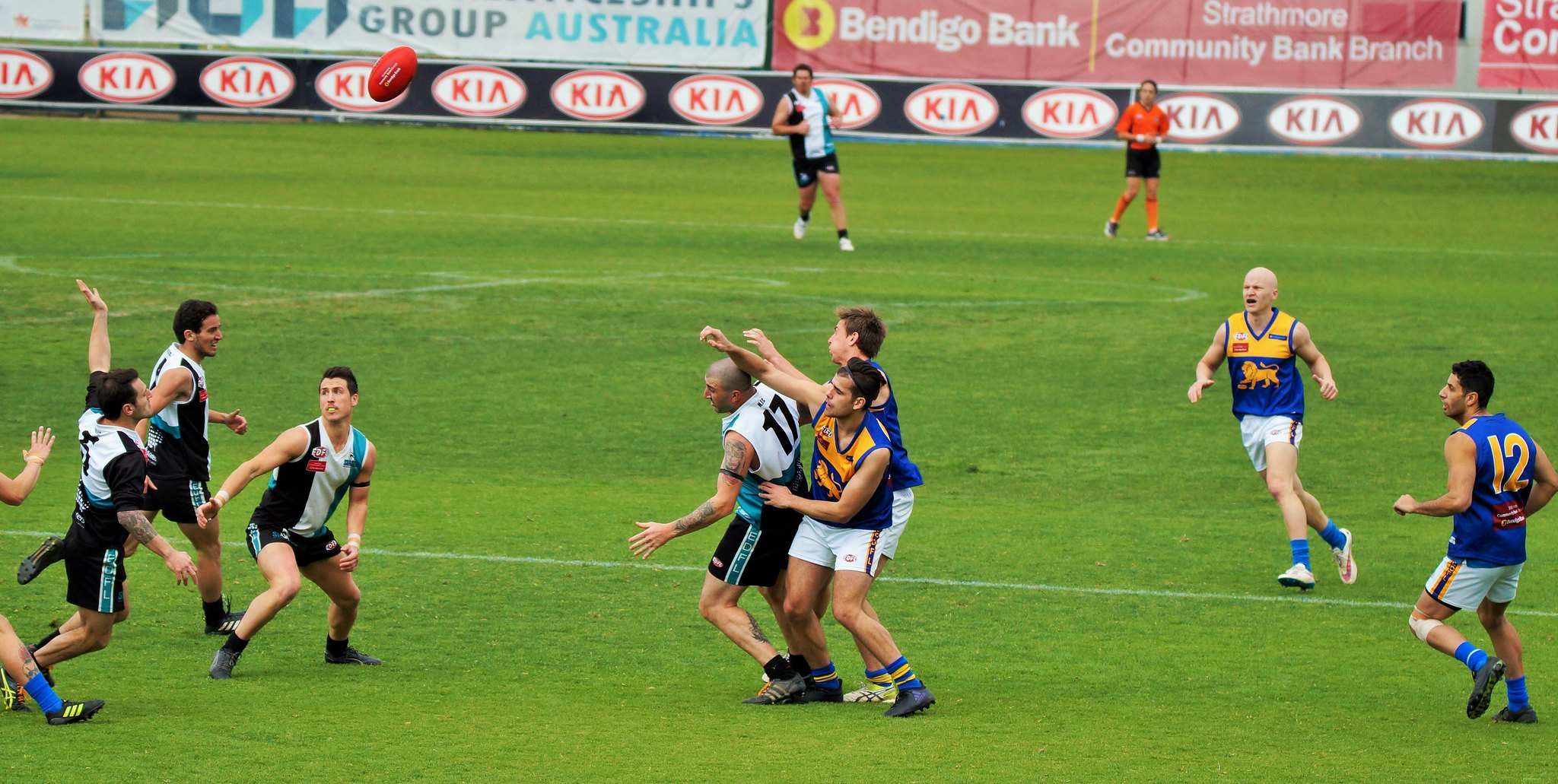The photograph captures a dynamic moment in a rugby game set on a lush green field extending into the distance. In the background, a series of advertisements line the boundary, including the prominent red-on-white KIA logo, along with ads for Group Australia, Bendigo Bank, and Strathmore Community Bank Branch. On the pitch, players from two distinct teams are intensely engaged. The first team dons blue and gold jerseys with a golden lion emblem on their midsection, paired with white shorts. The second team wears white and black jerseys with dark shorts. Central to the action, three players vie for dominance: two in blue and gold wrestling for position against a lone player in white and black, all contending for an incoming red rugby ball flying through the air. Additional players are dispersed across the field, some in mid-run with outstretched arms, and one player on the left appears to be falling, his arms splayed at a precarious angle. A referee in a red shirt, black shorts, and orange socks can also be spotted overseeing the chaotic play.